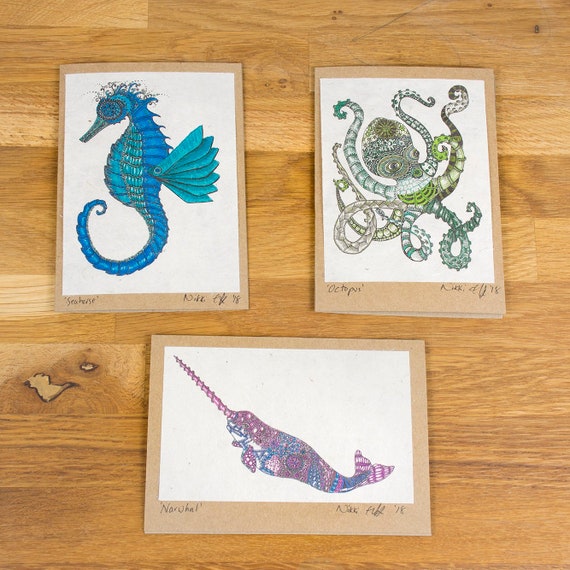A photograph captures a light oak table with horizontal planks, showcasing three pieces of handmade artwork arranged on it. The table holds two upright, portrait-oriented pieces at the top and one landscape-oriented piece at the bottom center. Each piece of art is set on a white background with a tan edge, resembling greeting cards on beige cardstock. 

On the upper left is a detailed depiction of a blue seahorse, facing left, with its tail elegantly curled. This seahorse is painted in various shades of blue—sky blue, teal blue, and a touch of sea green. Adjacent to it, on the upper right, is an intricate illustration of an octopus, rendered in a mix of green and gray hues. The octopus's many tentacles are gracefully curled around its head and underneath its body.

At the bottom center is an artwork of a swordfish, created with shades of blue and muted purple. The swordfish features a distinct, slender sword extending towards the top left corner, while its tail is positioned towards the lower right. The combined details of each piece highlight the artistic talent and vibrant use of color in these unique and expressive illustrations.